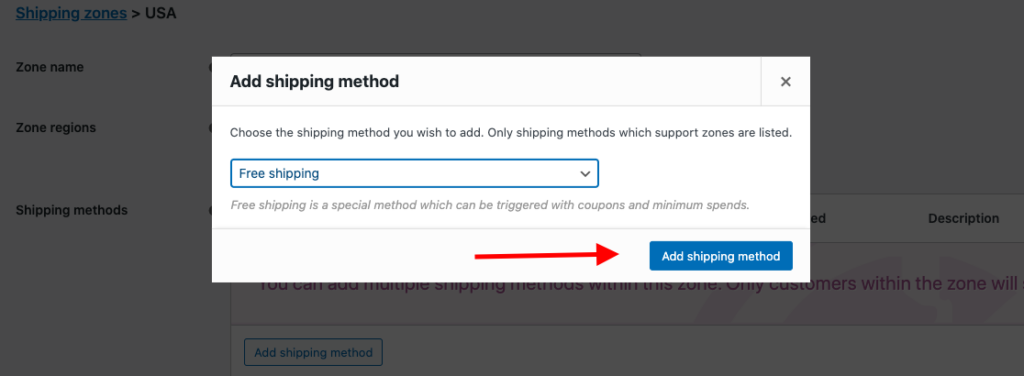This screenshot displays a section of a web page related to configuring shipping zones. A semi-transparent white overlay prominently takes up most of the screen, with a dark gray background visible beneath it. The gray background isn't interactive unless you engage with the white overlay.

On the dark gray background, the text "Shipping Zones" appears at the top in blue, followed by a forward arrow pointing to the right and the text "USA." Beneath this, several headings are listed: "Zone Name," "Zone Regions," "Shipping Methods," and a column displaying "Description" alongside an option to "Add Shipping Method."

The white overlay prominently features "Add Shipping Method" in bold black text at the top, followed by a smaller, lighter font instruction: "Choose the shipping method you wish to add. Only shipping methods which support zones are listed." Below this instruction is a drop-down menu defaulting to "Free Shipping." Accompanying this selection, a note in light gray italics provides additional information: "Free shipping is a special method which can be triggered with coupons and minimum spends."

Drawing attention to the bottom of the overlay, a red arrow points towards a dark blue button labeled "Add Shipping Method" in white font. The screenshot focuses exclusively on the shipping method configuration section, excluding broader elements such as the menu bar and the website's header or logo.